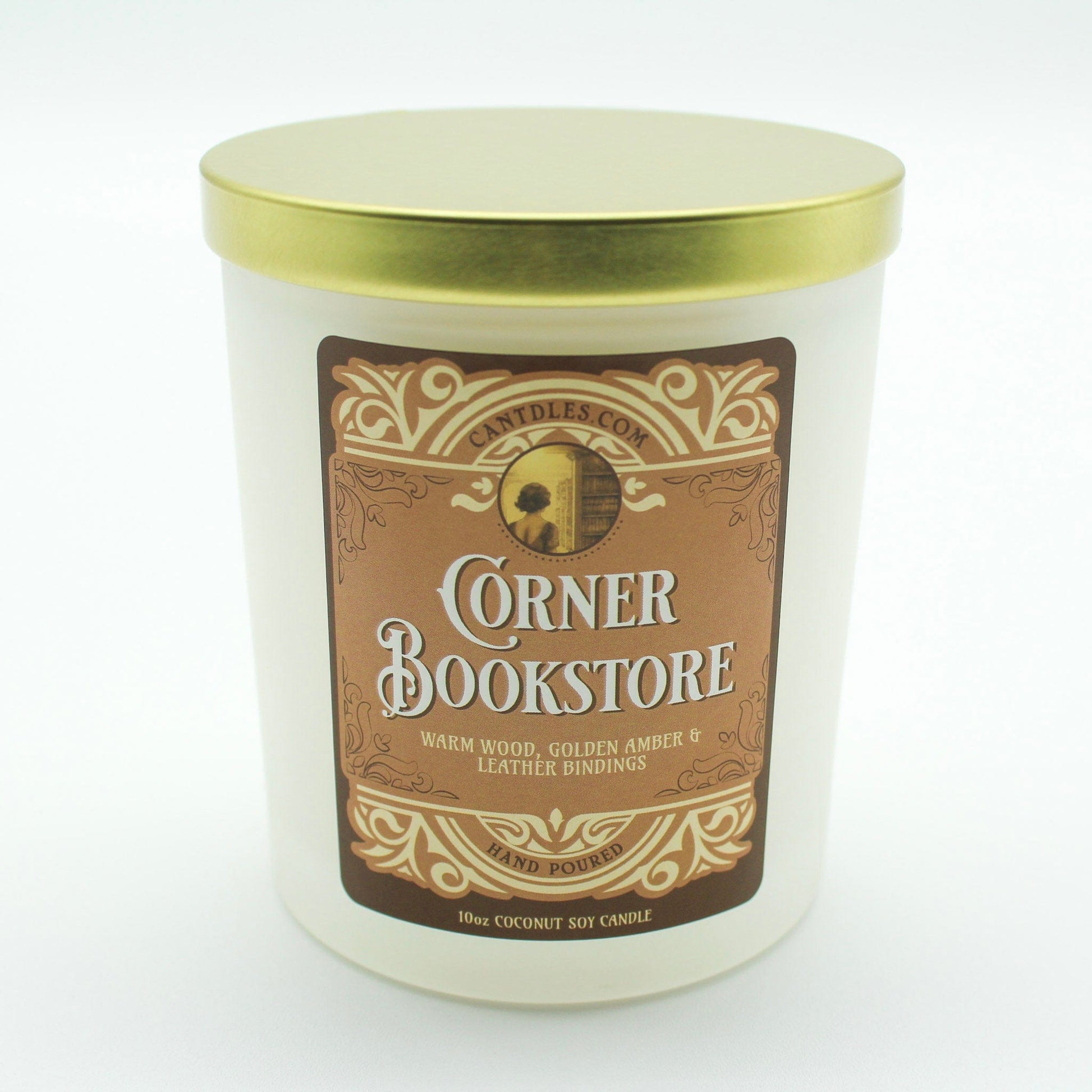This product image features a gift candle presented against a stark white background, with a slight shadow cast beneath it, emphasizing its centrality. The candle is housed in a frosted white glass jar topped with a gold metallic lid. Adorning the jar is a light brown and beige label with an antique, vintage-inspired design, mimicking carved wood with floral elements. The label features a small circular illustration of a woman gazing at a bookshelf, reminiscent of an old library scene. A URL, cantdles.com (C-A-N-T-D-L-E-S dot com), is prominently displayed at the top. The label’s centerpiece is the text "Corner Bookstore" in large, white, antique font with a dark brown drop shadow. Below this, it describes the candle’s scent profile: "Warm Wood, Golden Amber, and Leather Bindings.” Additional details at the bottom include “hand poured” in dark brown text and “10 ounce coconut soy candle” in beige text set against a dark brown border. This meticulous design evokes the cozy and nostalgic essence of a quaint bookstore.